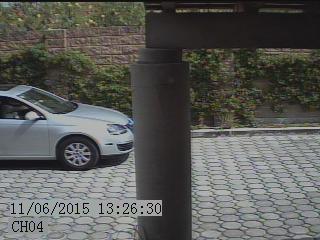The image, a rectangular screenshot from a security camera labeled as "CH-04", captures an entryway area on a clear, sunny day, dated 11-06-2015 at 13:26:30. Foremost in view is a cobblestone driveway composed of interlocking bricks, leading up to a prominent concrete column emerging from the bottom center of the frame. To the right, a sleek, silver sedan moves from left to right, with only its front half visible—no occupants discernible inside. In the background, a tall brick wall adorned with climbing vines and shrubbery stretches across the image, while further beyond, the terrain slopes with a mix of green bushes and yellowish plants, setting a picturesque backdrop.